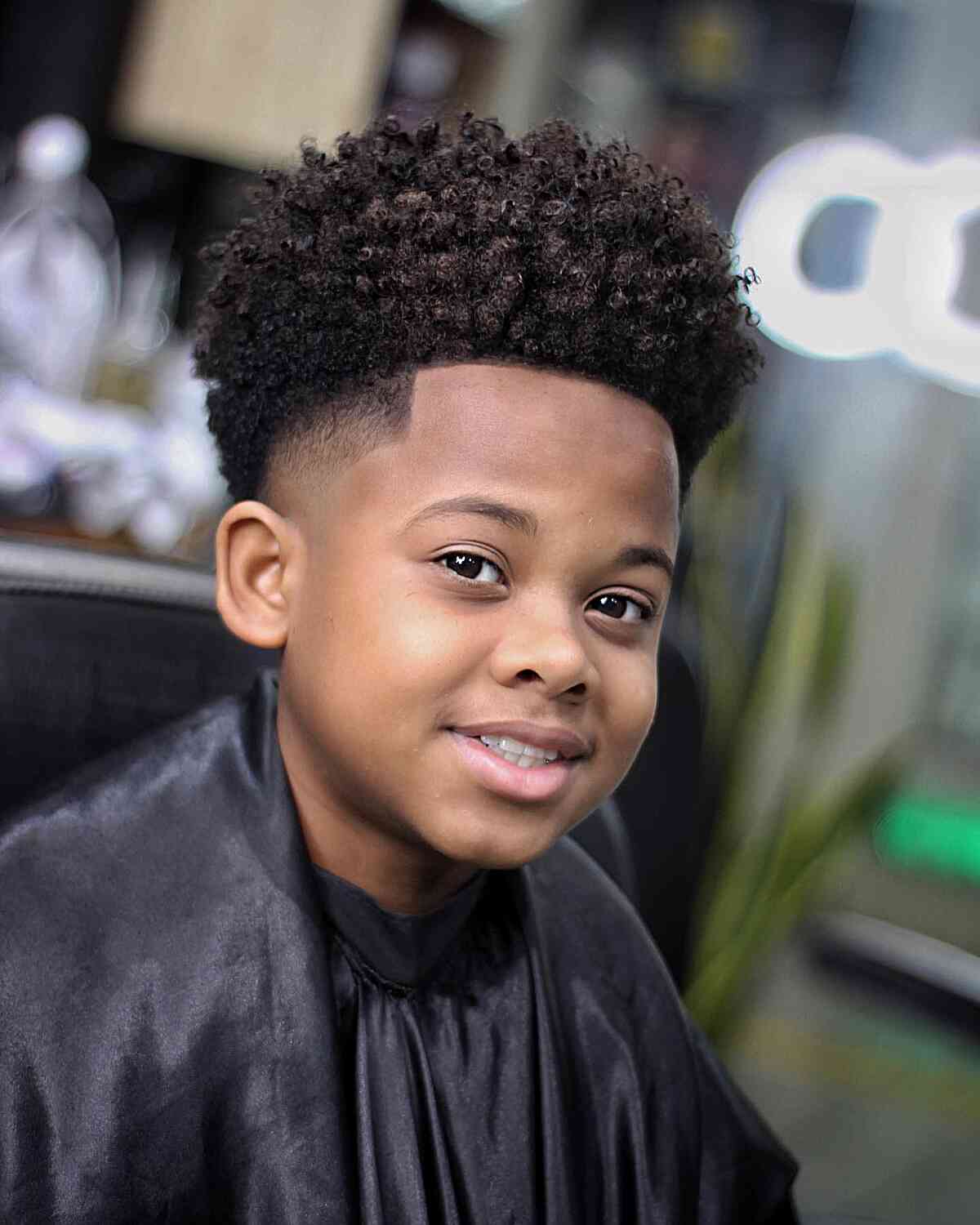The image portrays a cheerful young black boy, possibly around six or seven years old, sitting in a barbershop chair. He is wearing a black barbershop cape, suggesting he is either about to get a haircut or has just received one. His long, curly hair is styled high on top of his head, while the edges around the base of his skull are neatly faded. He has distinct facial features, including large, expressive brown eyes, wide nostrils, thick lips, chubby cheeks, bushy eyebrows, and somewhat prominent ears. He smiles brightly towards the camera, showcasing his very white teeth. The background is blurred but includes some indistinct elements like shelves, LED lights, perhaps a counter with glasses, and a curtain with a neon sign. Despite the blurred background, the boy is clearly the focal point of the image, standing out vividly.